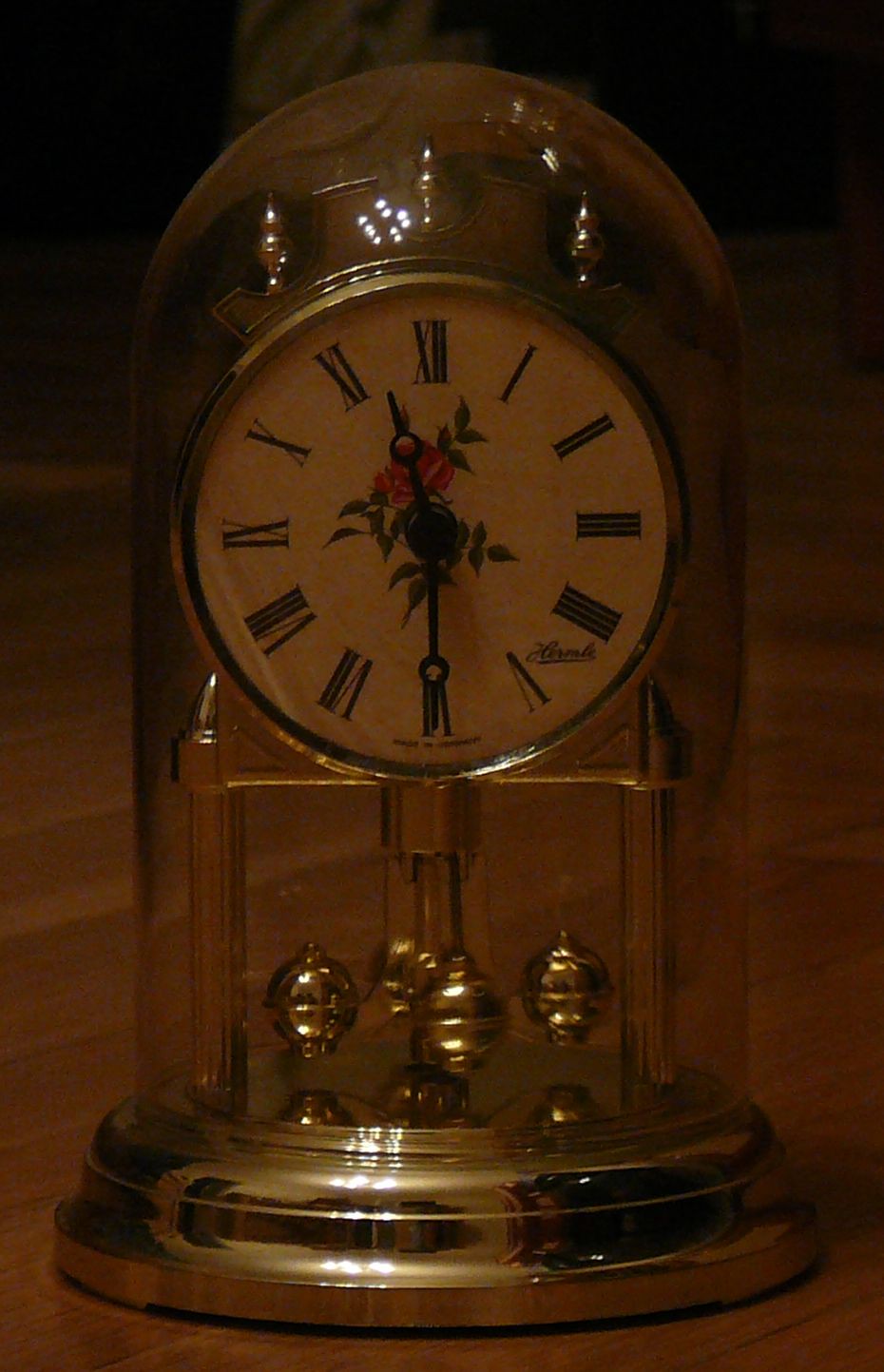The image features an antique-style clock encased in a glass dome. The base of the dome is crafted from a material that appears to be either chrome-plated gold or brass. This elegant clock stands on the base with three ornate legs, and directly beneath it, four gold balls are visible, designed to spin. The face of the clock is also adorned with gold and displays black Roman numerals. At the center of the clock face, there is an intricate illustration of a red rose encircled by green leaves. The clock hands are black and feature a distinctive circular design at their centers. The entire assembly rests on a table that appears to be made of either red oak or a lighter oak, contrasting against a stark black background. The image quality is notably grainy, contributing to the vintage feel of the scene.